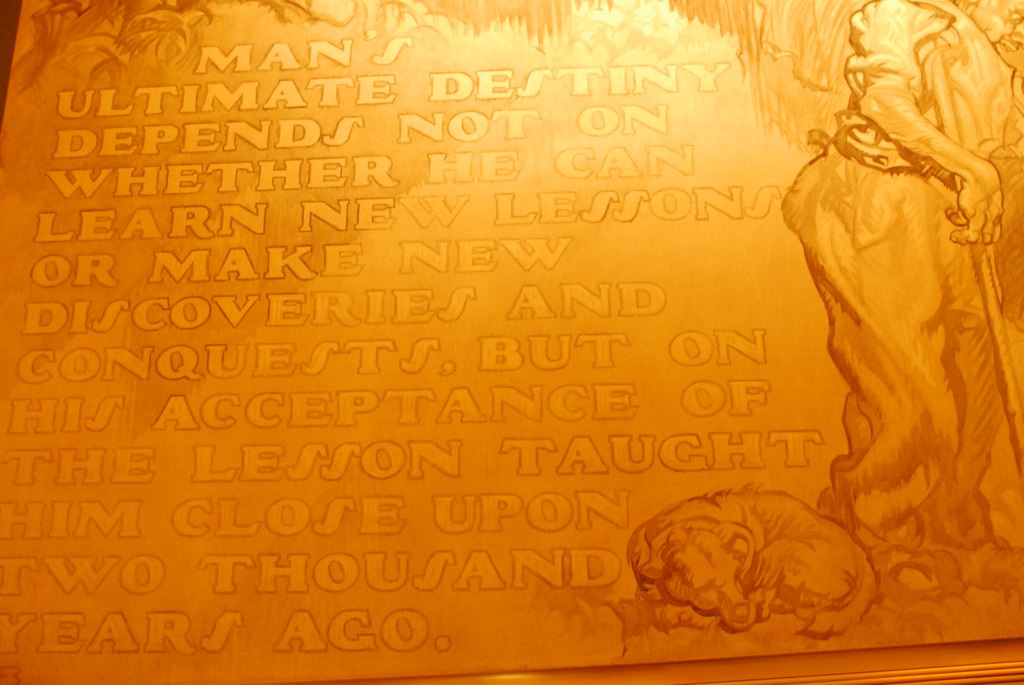The image shows a striking gold or yellow monochrome painting or drawing that radiates a shiny glow, especially at the top. On the right side, there is a detailed depiction of an old, possibly disabled person, hunched forward and draped in a dramatic, flowy robe, holding a cane in their right hand. The figure appears worn and is partly obscured, adding a sense of mystery and antiquity. At their feet lies a dog, possibly a golden retriever, curled up peacefully as if on a bed of clouds. The scene evokes a sense of serenity and contemplation. On the left side of the image, there is faint but distinct text that reads: "Man's ultimate destiny depends not on whether he can learn new lessons or make new discoveries and conquests, but on his acceptance of the lesson taught him close upon 2,000 years ago," potentially a reference to Jesus. The overall ambiance suggests the image could be part of a museum exhibit, illuminated thoughtfully by ceiling lights to highlight its reflective and introspective nature.